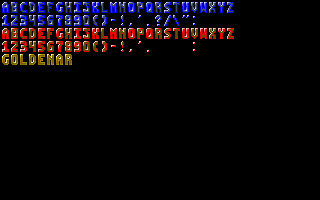The image displays a detailed font diagram on a small black square background, primarily concentrated in the upper left portion. The font style is blocky and somewhat hollow or grayish inside, providing a cartoon-like or game interface appearance. The visual layout starts with blue-colored characters from 'A' to 'Z', followed by numbers from '1' to '0', and includes various punctuation marks and brackets at the top. Directly below this array, there is a similar sequence in red with characters, numbers, and symbols mirroring the blue line above. At the bottom, the word "GoldenR" (possibly the name of the font) is prominently displayed in a golden hue. The bubble font gives a shiny impression, making the characters appear vibrant and dynamic against the stark black background.